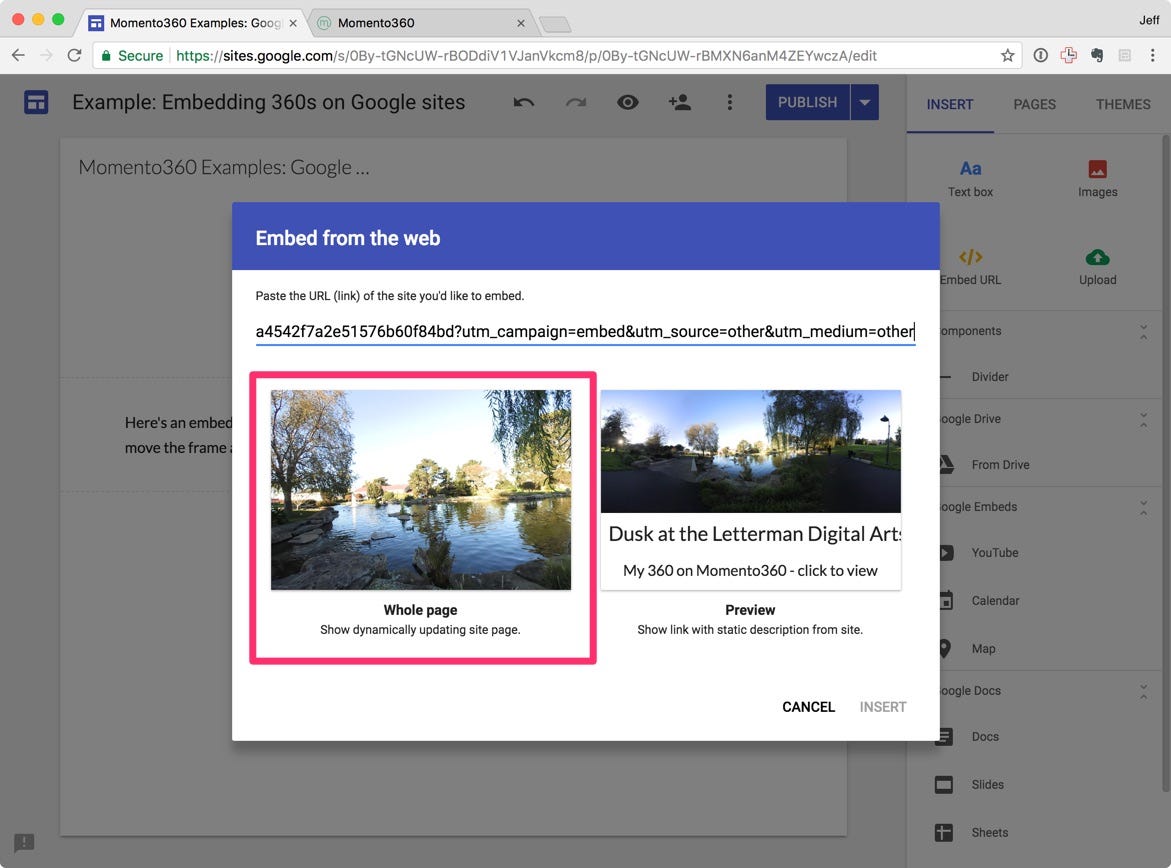The image displays a Chrome browser running on macOS, showcasing two open tabs. The active tab is set to sites.google.com, featuring a Google Docs document titled "Memento 360 Examples." Much of the document's content is obscured by a pop-up window labeled "Embed from the web." This pop-up prompts the user to paste the URL link of the site they'd like to embed. The interface offers two options: "Whole Page," which shows a dynamically updating site page, and "Preview," which displays a static description of the site. A long URL is visible within the input field of the pop-up. In the background, partially hidden by the pop-up, is a prominent blue "Publish" button, hinting that the user is in the process of embedding content into the document.